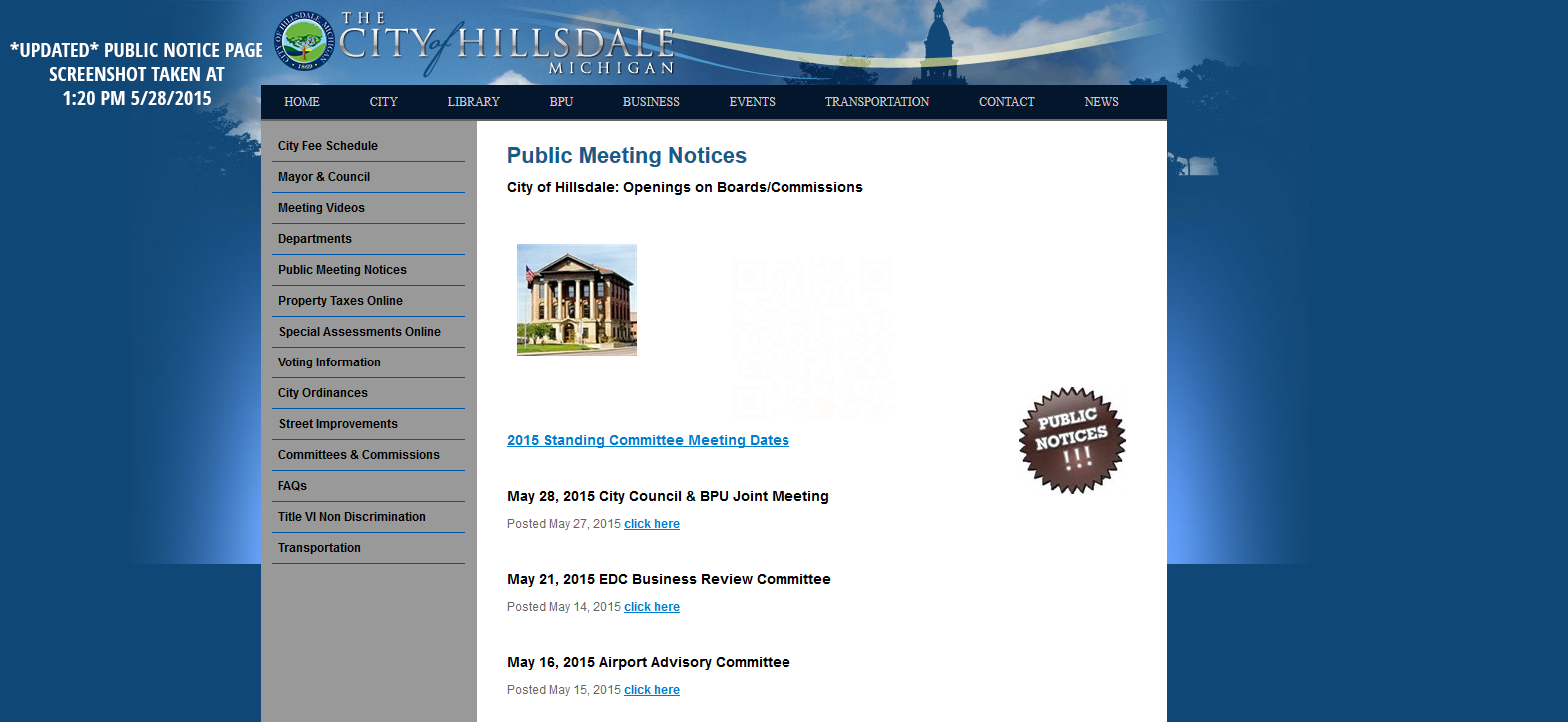Sure, here’s a cleaned-up and detailed description of the image:

Top left corner: A timestamped text reads "Updated Public Notice Page" with a screenshot taken at 1:20 p.m. on May 28, 2015. 
Top section: "Hillside" is mentioned, indicating the place as Hillsdale, Michigan, written in silver text on the right. 
Adjacent to this, a blue logo featuring a green tree is visible.
Towards the bottom: Tabs are displayed in white on a black background. Starting from the top left of the main page, the tabs are: Home, City Library, PPU, Businesses, Events, Transportation, Conduct, and News.
Top right corner: On the left side of the main page, there’s a vertical side menu with text written in black, items separated by blue lines. The menu items include:
- City Fee Schedule
- Mayor and Council
- Meeting Videos
- Department Public Meeting Notice
- Property Tax Online
- Special Assessment Online Voting Information
- City Ordinances
- Streets Improvement Committee and Commissioned Effects
- Title VI Non-discrimination and Lastly Transformation

Bottom left section: A blue text title reads "Public Meeting Notice." Below this, in black text, it says "Seat Office Date Openings on Board or Commission." An image of a building, brown in color, is displayed below this text.
Further down: Blue text reads "2015 Standing Committee Meeting Dates" with specific dates in black text except for a clickable "Click Here" in blue. Meetings listed are:
- May 28, 2015: City Council and PPU Joint Meeting (posted May 27, 2015) [Click Here]
- May 21, 2015: EDC Business Review Committee (posted May 13, 2015) [Click Here]
- May 16, 2015: Airport Advisory Committee (posted May 15, 2015) [Click Here]

Right side: A brown stick with the text "Public Notices" is visible, set against a white background. The overall background of the image is blue with some trees visible on the right side.